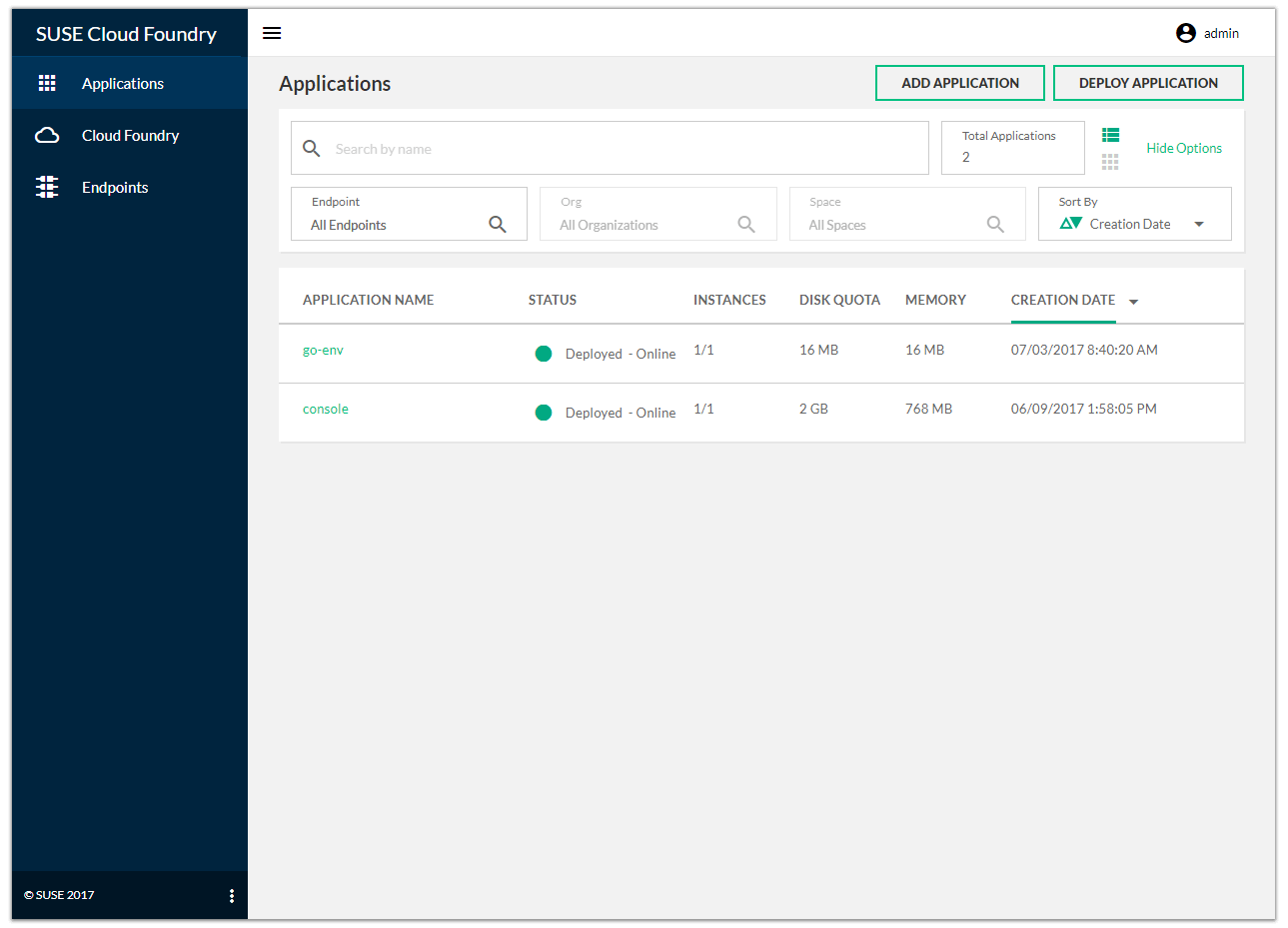The image features a screenshot of a SUSC Cloud Foundry web interface. The interface consists of several sections and panels with a distinct color scheme and organizational layout:

On the top-left side, the heading "SUSC Cloud Foundry" is prominently displayed. Below this heading, there are three navigation categories labeled in white text: "Applications," "Cloud Foundry," and "Endpoints," arranged vertically. The sidebar housing these categories has a dark bluish-gray background. At the very bottom of this sidebar, there is a small section with a black background displaying the text "2017."

The central and right portions of the image are primarily light gray, with the top segment being white. In the top-right corner, there is an "Admin" label accompanied by a profile picture, indicating the user management section.

Under the main heading, the interface offers options such as "Applications," "Add Application," and "Deploy Application," highlighted with a green rectangular border. Beneath these options, a search bar invites users to "search the name," followed by the label "Total Applications."

Further down, the interface displays an "Endpoint" section followed by two additional categories labeled "Org" and "All Organizations," and "Space" and "All Spaces," respectively. To the right, there is a sorting button labeled "Sort by Creation Date."

The primary table's column headers list the following categories: "Application Names," "Status," "Instances," "Quota," "Memory," and "Creation Date." Below these headers, the actual data for applications is presented in rows, with each column filled accordingly from left to right, maintaining the light gray background of the table.

Overall, the image captures the comprehensive layout and design of the SUSC Cloud Foundry web interface, with clear, well-organized sections delineated by color and functional grouping.